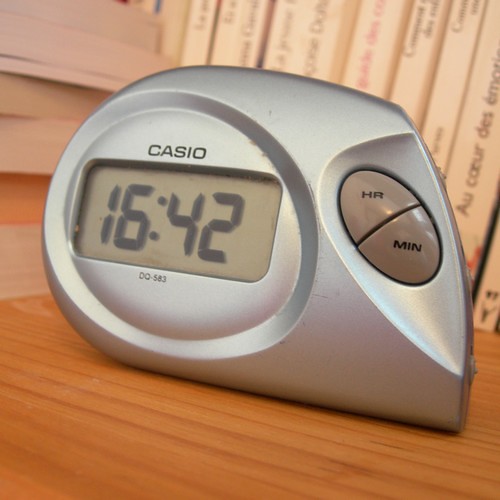This image features a close-up of a Casio digital alarm clock resting on a light stained wooden desk or nightstand. The clock has a unique, modern design with a silver plastic body, resembling a shape close to a rhombus with one side curved. The digital display reads "1642," indicating military time which suggests the setting is possibly in Europe. Below the display, the model number "DQ-583" is faintly visible. To the right of the display, there are two buttons labeled "HR" for hour and "MIN" for minute, used to adjust the time. In the background, there is a stack of books lying horizontally with only their pages visible, characterized by their white or ivory color. Behind this stack stands a row of vertically aligned books with readable spines, written in French, pointing to a possibly European scene. The overall composition creates a harmonious blend of modern technology and traditional wooden aesthetics, set against a backdrop of literary culture.